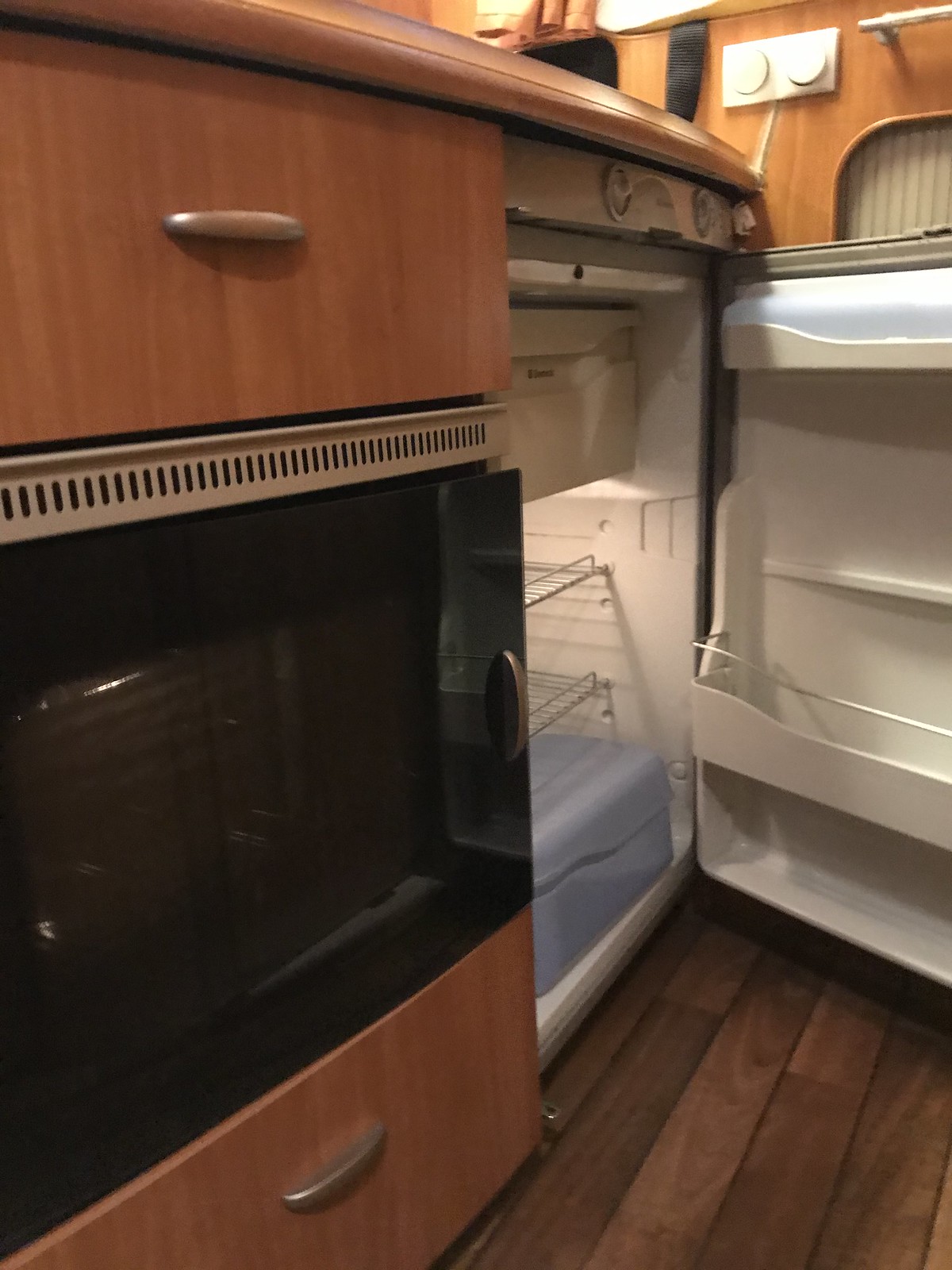In the kitchen area of an RV or camper, a compact, real-life photograph captures a mini-fridge with its door ajar, light illuminating its pristine white interior. The refrigerator, featuring two white wire racks and a small freezer compartment at the top, sits empty. It is nestled into a warm, brown-orange wooden recess beneath a flat surface, possibly a countertop or bar area. Adjacent to the fridge, and encased in the same wooden cabinetry, is a black microwave with a sleek silver handle and a shiny black glass door. Above the microwave is a silver vent, complementing the two sleek, modern drawers that provide a functional, streamlined appearance. The floor beneath is made of dark brown hardwood, displaying tongue and groove craftsmanship, contributing to the cozy and stylish interior.